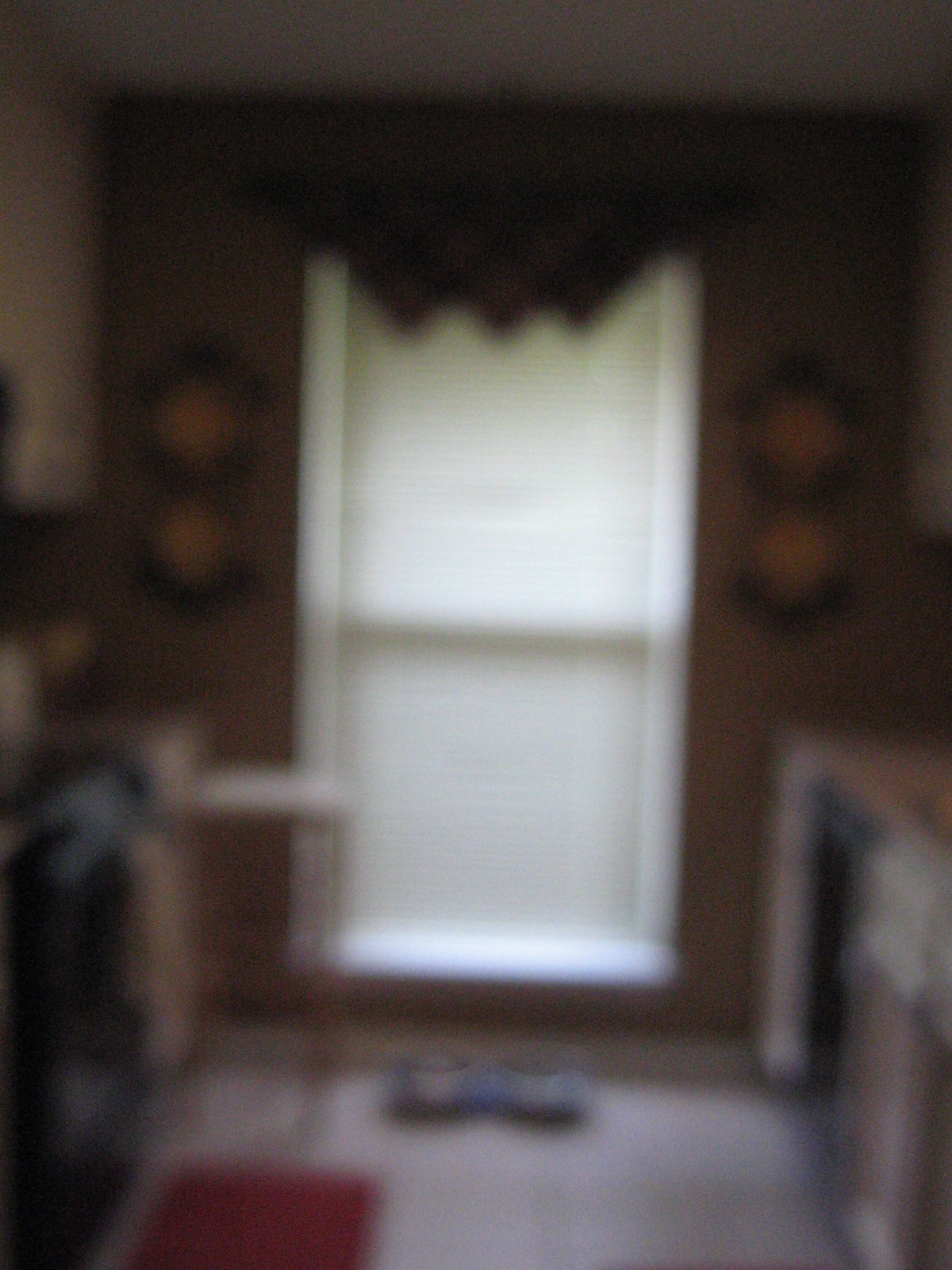A blurry and grainy photo captures the interior of a vintage-styled kitchen, evoking design elements from the 1970s to early 1990s. On the left side, a stove is accompanied by a pull-out cutting area just beside it. Adjacent to these is what seems to be a sink and a dishwasher. The focal point of the image is a large window that almost reaches from the floor to the ceiling, framed by a decorative valance at the top and flanked by additional adornments. The window’s blinds are closed, casting a dim light throughout the room. On the floor, a placemat or mat with bowls likely intended for a pet’s food and water is visible. In front of the stove lies a red rug. The entire scene is shrouded in darkness, contributing to the overall impression of an era-specific aesthetic.